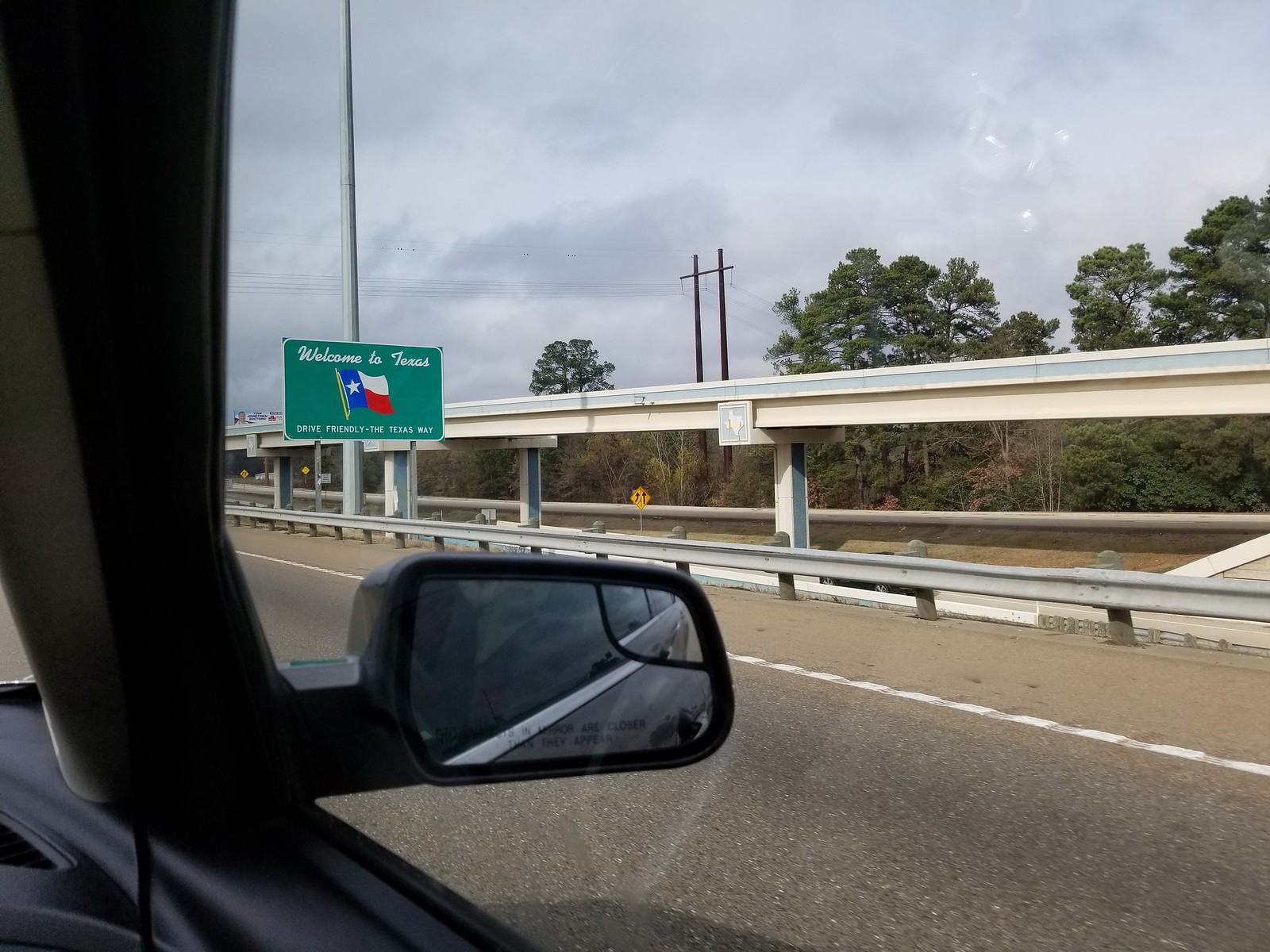This photograph captures the moment a driver is cruising down the interstate, taken from the perspective of the passenger-side window. In the foreground, a solid metal guardrail runs parallel to the highway. A prominent green sign on the left side of the guardrail warmly greets newcomers with "Welcome to Texas," accompanied by a vivid depiction of the Texas state flag featuring its iconic blue vertical stripe with a white star and horizontal white and red stripes. Below the flag, partially visible text suggests driving guidance typical in Texas.

To the right of the interstate, a substantial overpass bridge soars in the background, serving as a distant focal point. Nearby, two tall wooden electrical poles, connected by a wooden crossbeam, stand sentinel among a cluster of trees. Further enhancing the scene, a diamond-shaped road sign displays clear directional arrows: one pointing straight ahead and another curving to the left, guiding travelers on their journey. The car’s sleek black interior frames this quintessential Texan landscape, encapsulating a slice of life on the road.